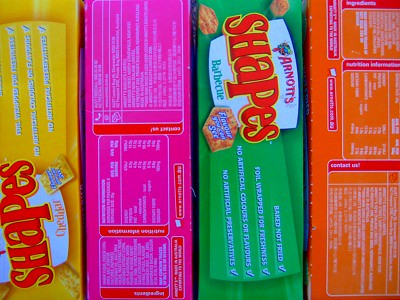In the image, there are four vertically standing boxes viewed from above, each distinct in color and design. Starting from the left, the first box is yellow with a red brand name printed on a white background, though only one edge of this box is visible. Moving to the right, the second box is pink, featuring numerous small paragraphs of white text interspersed with red labels. Next, the third box is green, prominently displaying the product name "SHAPES Barbecue" with "Arnott's" in pink, "SHAPES" in red and yellow, and "Barbecue" in blue on a white background. Finally, the fourth box is orange and, similar to the pink box, covered in an array of small white text accompanied by red labels.